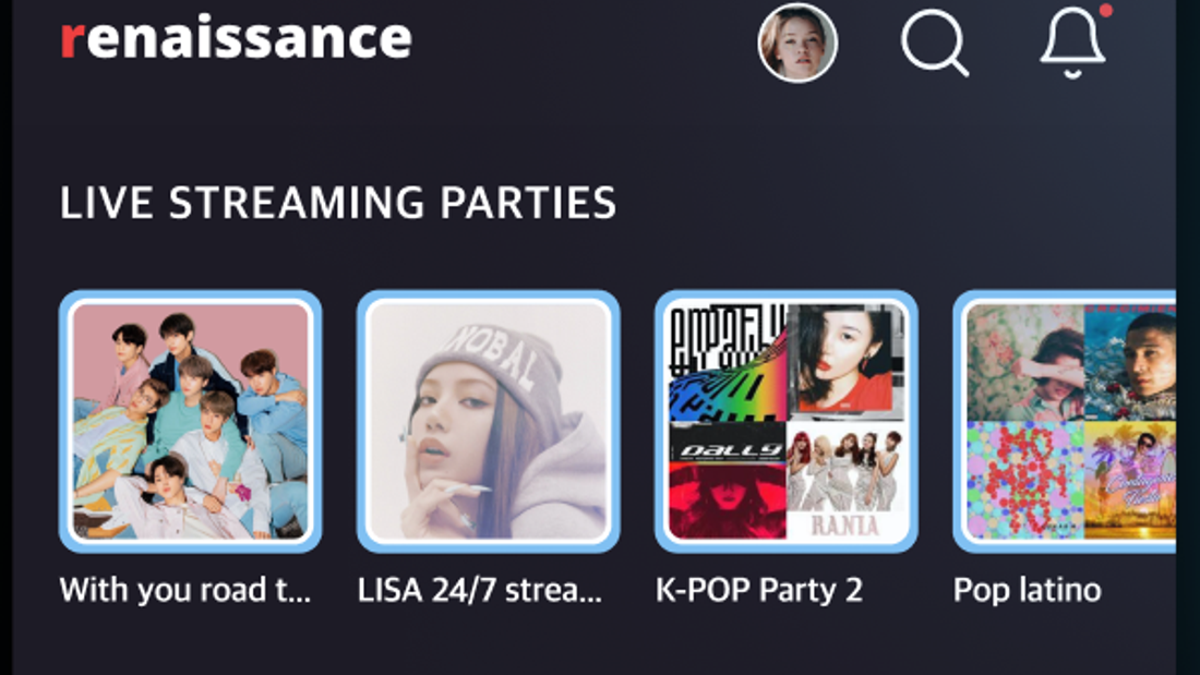**Caption for the Website Home Page Image:**

At the top of the website's homepage, prominently displayed is the site name "Renaissance," with a red 'R' and the remaining letters in white. Adjacent to the website name, on the right side, is a user's profile picture featuring a young woman of European descent. To the right of her image, there is a magnifying glass icon symbolizing the search function, followed by a notifications bell, which has a red dot indicating one new notification.

Beneath this header, in white text, are the words "Live Streaming Parties," accompanied by a series of photograph icons showcasing various young individuals. The first photograph features a group of Asian teenagers or tweens, possibly a K-pop band, captured in a relaxed, casual pose. The only visible letters in their caption are "With you road, T and an S..."

The second photograph depicts a young woman of Asian descent wearing a wool cap. The visible letters in her caption read "N-O-B-A-L." She strikes a slightly sensual pose with her finger near her mouth, her long hair framing a hooded sweatshirt, and her long fingernails adding to her stylish appearance.

The third photograph appears to be of a possible band named "Rainia." The visible letters indicate "Ranta" and "DALG" (possibly "D-A-L-L" or "D-A-L-L-G"). It showcases young women dressed in satin, form-fitting dresses or gowns.

The final photograph labeled as "Momento" (M-O-M-E-N-T-O) features a young man looking directly at the camera, while a young woman beside him appears to be shyly hiding her face.

This homepage layout combines the social interaction component with visual elements that highlight the platform's vibrant and youthful community.